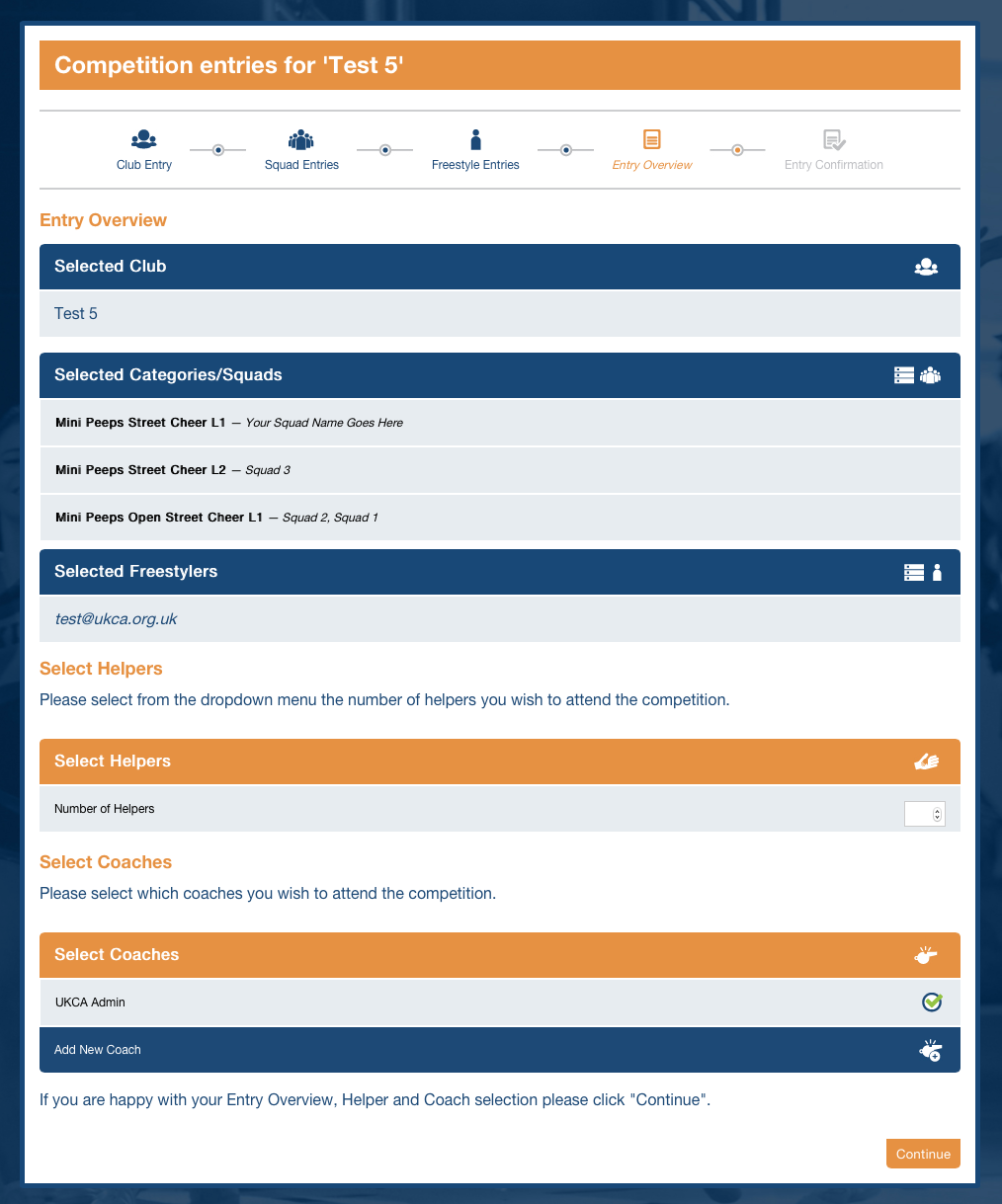The image displays a screen with a white background, framed by a dark blue border. At the top, there's an orange bar with white text that reads "Competition Entries for Test 5." Below the orange bar, blue and orange text accompanied by small icons are visible. 

Next, an orange heading labeled "Entry Overview" appears. Beneath it, a dark blue line contains white text stating "Selected Club." Below this, a section with a light blue background displays "Test 5" written in dark blue text. Further down is a blue background section labeled "Selected Categories/Squads" in white text. 

Although there is some dark, small, and blurry text beneath this section, it remains unreadable. Additional lines in dark blue and gray, with differently colored text, are also present. At the bottom of the screen, there is a small orange button with white text that says "Continue." Above this button, on a white background, light blue text advises, "If you are happy with your Entry Overview, Helper, and Coach Selection, please click Continue."